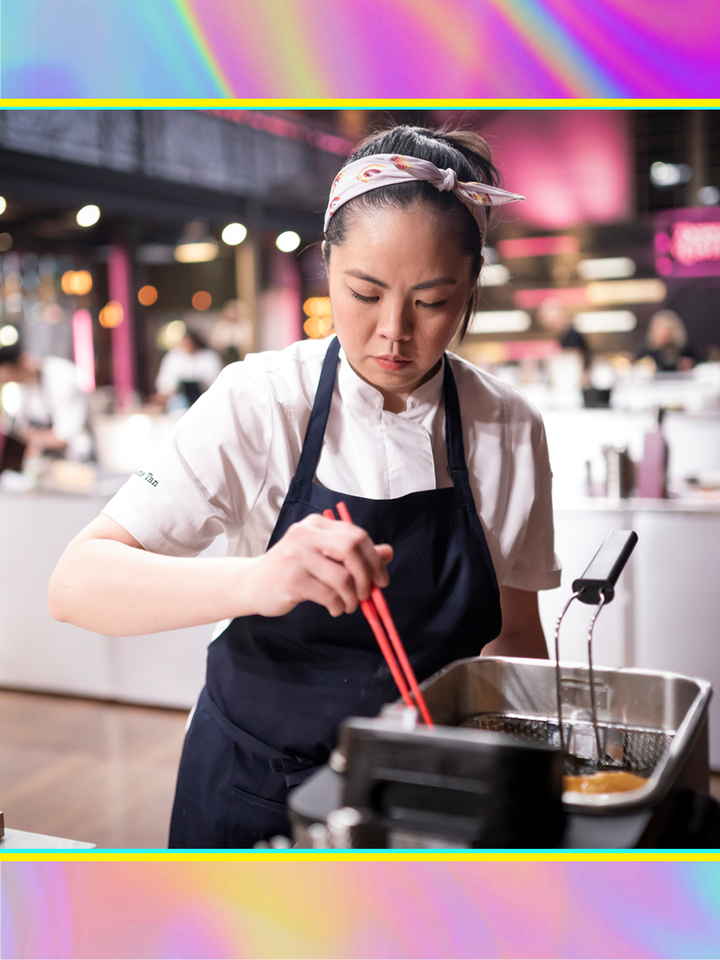This image is a vertically aligned rectangle bordered by thick, multi-colored bands featuring blue, yellow, purple, and pink tie-dye. Within these borders, a horizontal yellow line runs just above the bottom edge. At the center, a square photograph captures a scene of a focused Asian woman, possibly a chef, in the midst of cooking. Her hair is tied back in a ponytail and adorned with a white scarf decorated with red designs, knotted at the top. 

She is intently looking down at a large metal fryer tray, where a food item is being cooked. A thermometer is visible protruding from the tray, indicating she's closely monitoring the temperature. The woman holds orange chopsticks in her right hand and has a navy blue apron over her white button-down shirt with a black print on her right sleeve. Her left arm rests at her side. The background appears blurred, but you can make out other chefs busy at white-colored counters, suggesting the setting is a bustling restaurant kitchen.